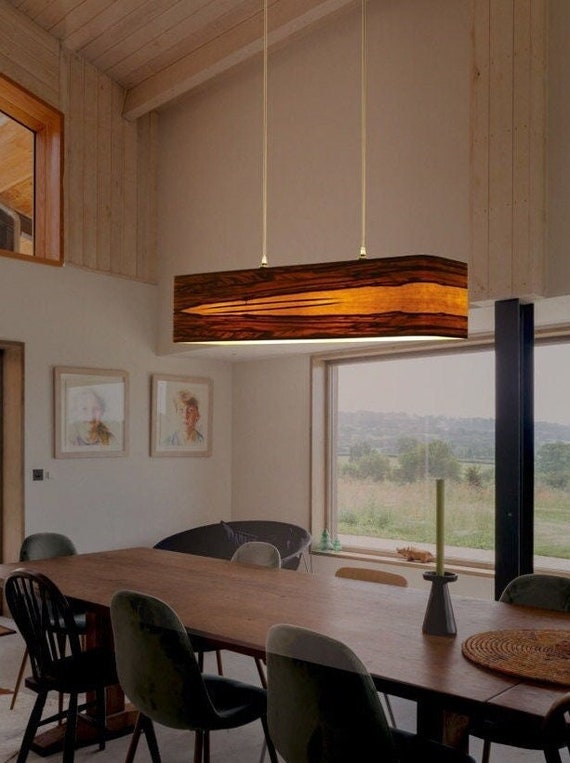This image captures the interior of a dining room, which appears staged as though it is part of a real estate listing or rental advertisement. The room features a long, somewhat dated wooden dining table, reminiscent of designs from the 1980s. Surrounding the table are various chairs, including one with a wooden back and others with plastic backs, emphasizing a mismatched style.

On the table, there's an arrangement that includes a distinctive long candlestick in an army green candle holder and a woven wicker table setting ideal for a hot plate. The surrounding décor includes a couple of pictures on the cream-colored walls. Prominent in the room's design is an overhead chandelier with a brown exterior and two gold chains affixed to the ceiling, which has light-colored, almost pinkish wood rafters.

The dining room is notably spacious with high ceilings, featuring light brown wood rafters that add to its rustic charm. The floor appears to be either gray linoleum or cement, contributing to the room’s vintage aesthetic. A window reveals an expansive outdoor scene with a mountainous background, numerous trees, and a vast grassy area, suggesting the home is situated on a large, secluded property. Additionally, a smaller window in the upper corner and a doorway at the bottom lead to other parts of the house. The overall feel is one of a dated but charming dining area with a blend of eclectic and nostalgic elements.